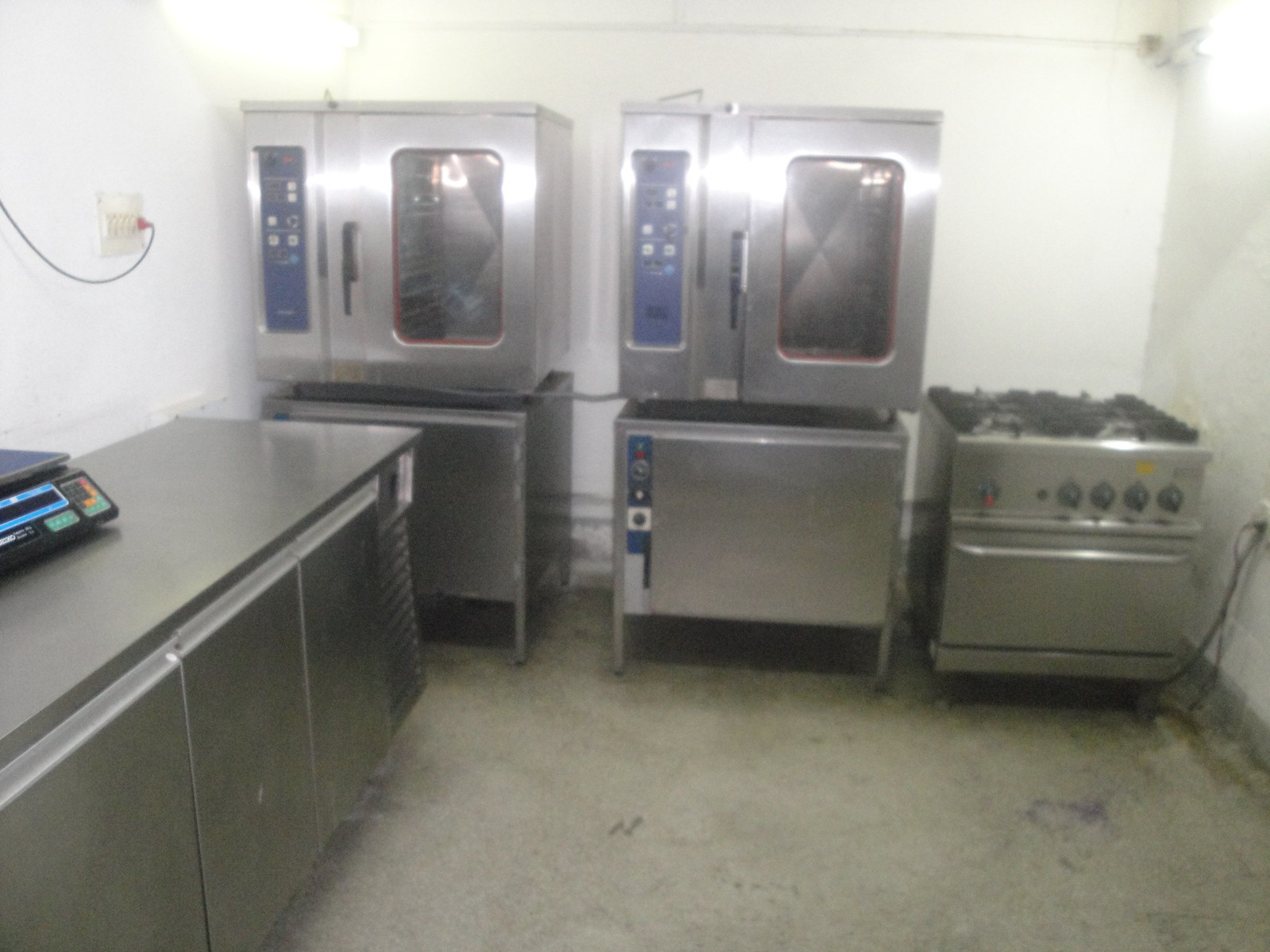This image was captured indoors in a rather industrial-looking kitchen. The scene is set against a backdrop of white walls and a dingy, scuffed floor. In the top left corner, there is a light source providing partial illumination over a suite of gleaming stainless steel appliances that dominate the space. Center stage are two large, industrial-grade ovens or rotisserie cabinets, sporting large clear panels on the right side and control panels on the left. Adjacent to these is an imposing stainless-steel gas hob and oven combination. A metallic work surface extends along the side wall, beneath which is a storage cabinet of the same shiny finish. At the forefront, there is another stainless steel unit with an industrial-grade scale on top of it; the scale is mainly black with colorful red, green, and blue buttons. The overall scene is enhanced by the presence of an electrical outlet with something plugged into it, although the image quality is somewhat grainy, making finer details harder to discern.